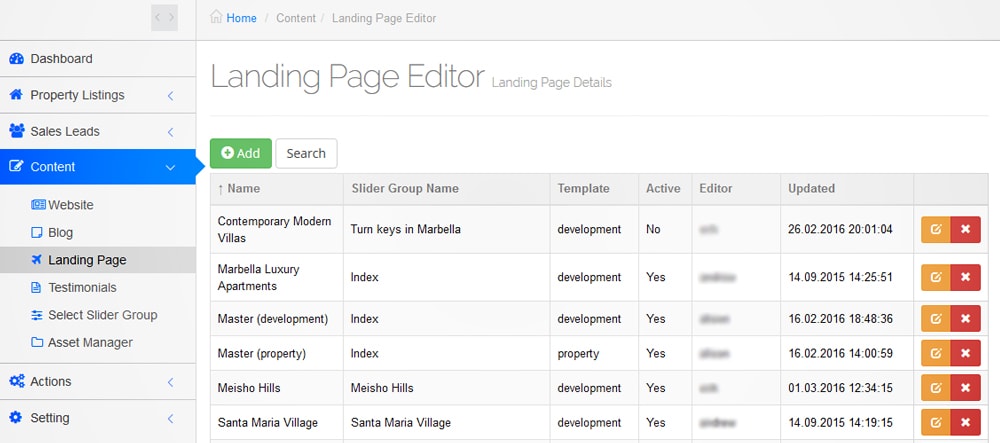The image depicts a detailed dashboard interface for a property management system, filled with various elements and functionalities. At the top, there is a grey header featuring navigational arrows inside a darker grey box. Below the header, the interface is predominantly blue with an icon of a house accompanied by the word "Home."

The left-hand side features a vertical menu with several items:
- **Dashboard**
- **Property Listings**
- **Sales Pending**
- **Leads**

These are followed by further categorized sections:
- In blue text on a white background: **Content**
- In white text on a grey background: **Webpage** and **Blog**
- In grey text on a black background: **Landing Page**
- In white text on a grey background: **Testimonials**, **Select**, **Slider Group**, **Asset Manager**, and finally **Actions and Settings**.

On the right-hand side, the interface leads into a form for the **Landing Page Editor** with corresponding details. Notably, a blue button labeled "Add" is shown prominently. Below it, a white button on a black background labeled "Search" is present.

Further down, a grey section lists various properties with columns such as "Name," "Slider Group Name," "Template," "Active," "Editor," and "Updated." 
There are six entries listed:
1. Contemporary Modern Villas
2. Mabel Luxury Apartments
3. Master
4. Master Property
5. Machino Hills
6. Santa Maria Village

All entries are marked as "Active" except for the "Contemporary Modern Villas," and the update timestamps range from 2015 to 2016, indicating that this screenshot is relatively old.